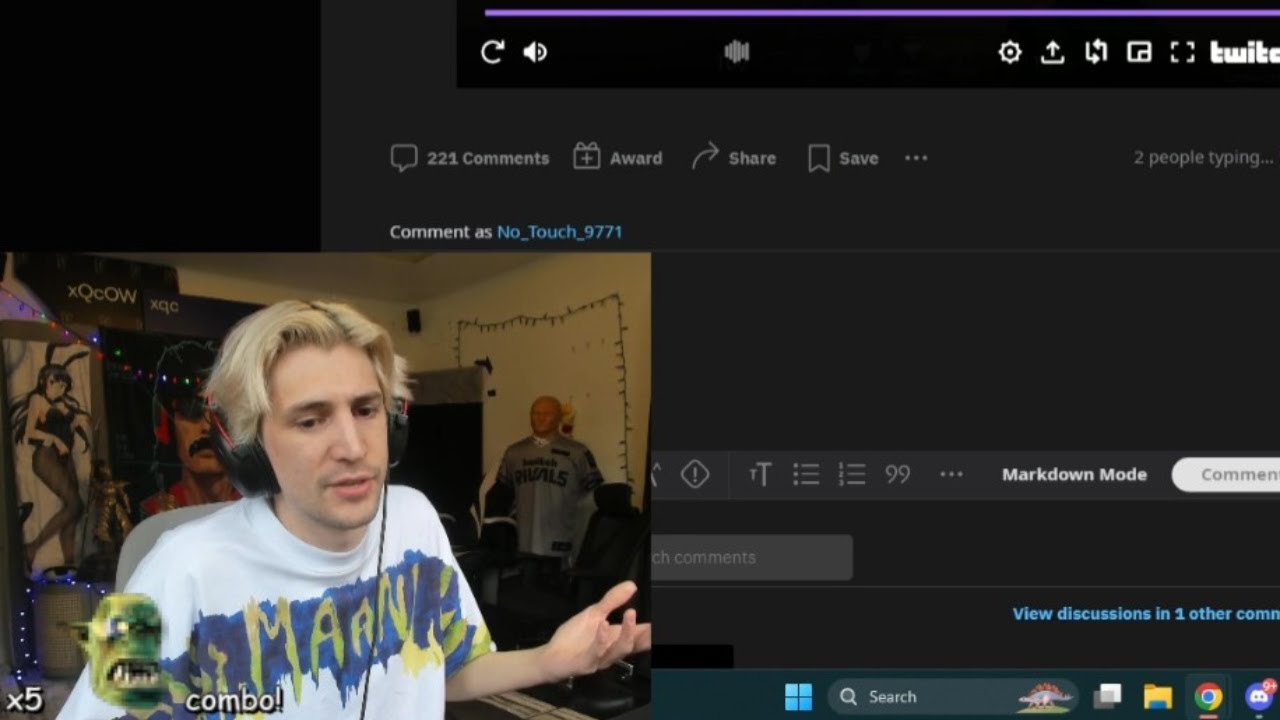A screenshot captures a user's web browser displaying the familiar interface of Google Chrome, identifiable by the emblem located at the bottom right of the image. The user has two instances of Chrome open, alongside a persistent Discord notification indicating 9+ unread messages.

The focal point of the browser is a Reddit page, distinguished by characteristic features such as the comment button, award option, share/save buttons, and the ellipses for additional options. The user’s Reddit profile is clearly visible as 'Notouch9771', with an indication that two users are currently typing.

Central to the screenshot is an embedded Twitch clip, showcasing a notable streamer, XQC. This clip appears to have already been watched, as evidenced by the visible restart icon in the top-left corner of the Twitch player. Additional Twitch player controls, such as mute sound, open Twitch, settings, and full-screen options, are also prominently displayed. The video of the streamer, minimized to the bottom-left corner of the screen, suggests that the user is simultaneously watching the stream while browsing Reddit.

This richly detailed capture illustrates the multitasking nature of the user's online activity, seamlessly blending social media interaction, community engagement, and live-streamed entertainment.